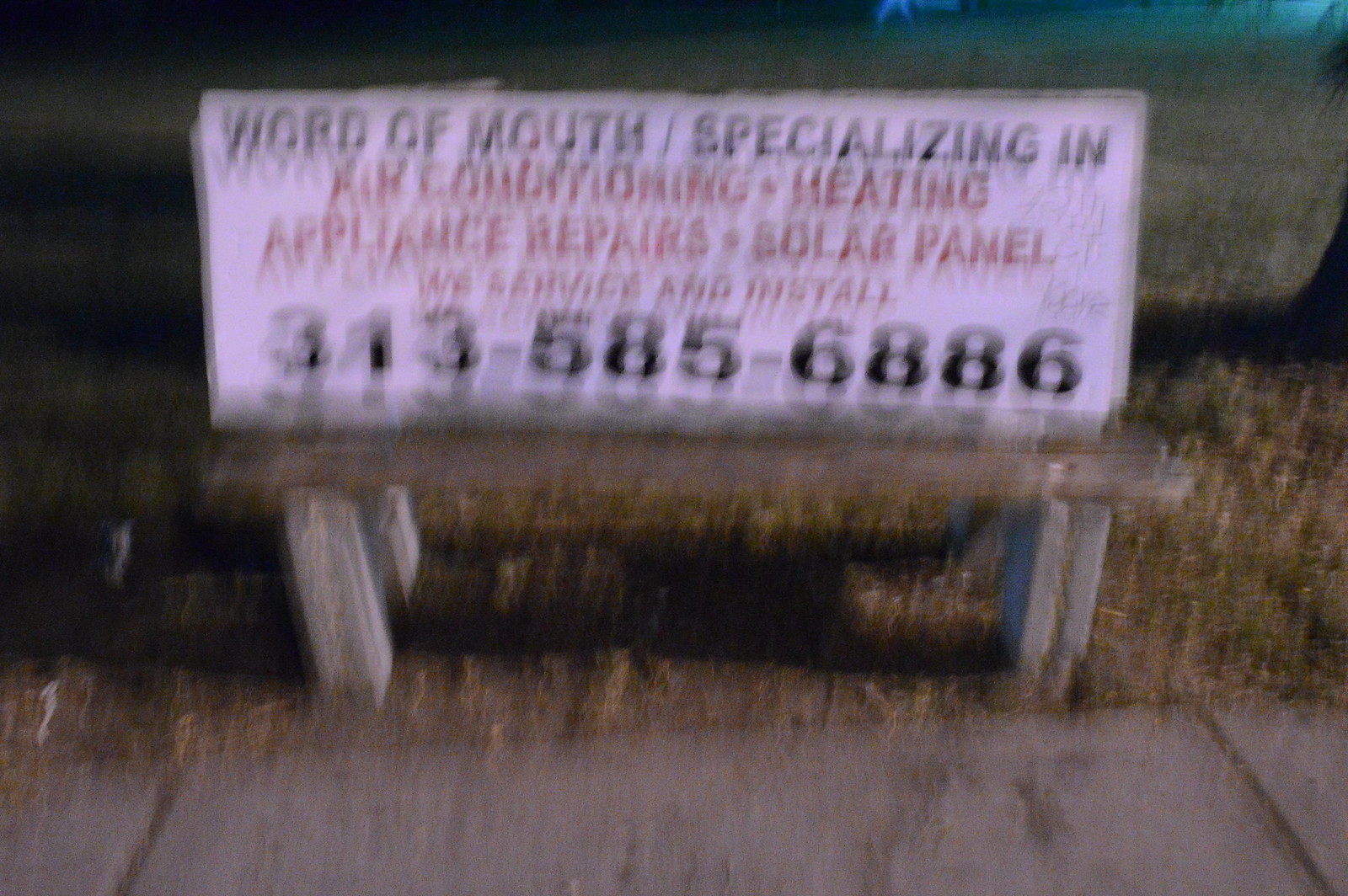The photograph is severely out of focus, yet some details can still be discerned. At the bottom of the image, a segmented sidewalk is visible, with clear lines dividing its sections. Adjacent to the sidewalk stands a wooden bench secured with concrete legs. Affixed to the back of the bench is an advertisement sign that reads: "Word of Mouth: Specializing in Air Conditioning, Heating, Appliance Repairs, Solar Panels. We service and install. 313-585-6886." Surrounding the bench is a patch of brown, dried-up grass, indicative of neglect or drought. To the right of the bench, a tree trunk emerges from the ground, casting a shadow that stretches out towards the left.